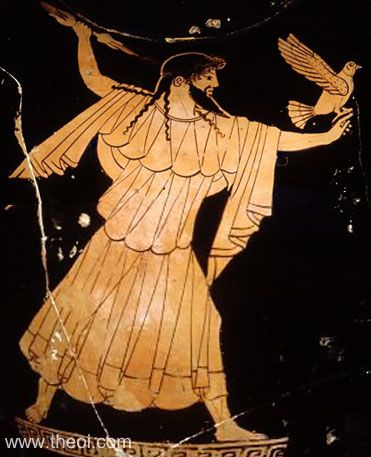This rectangular image, set against a black background marred with white spots and streaks, depicts an intricately detailed painting that suggests a religious or mythological theme. The central figure is a bearded man with long, curly hair ending in braids, and a pointed beard, possibly representing a biblical or ancient mythological character. He wears a long, flowing robe and stands on what might be a stage or an altar. His left arm is extended forward, his wrist slightly curved upwards with a bird, possibly a symbol of peace or divinity, perched on his finger. Meanwhile, his right arm is raised behind him, clutching a spear that hints at a dramatic narrative moment, possibly a sacrificial act or a moment of divine judgment. The entire composition is rendered primarily in shades of brown and black, and the artwork includes the URL www.theol.com at the bottom, indicating its photographical reproduction. The damaged appearance, with visible cracks, implies that the original piece might be aged and cherished.